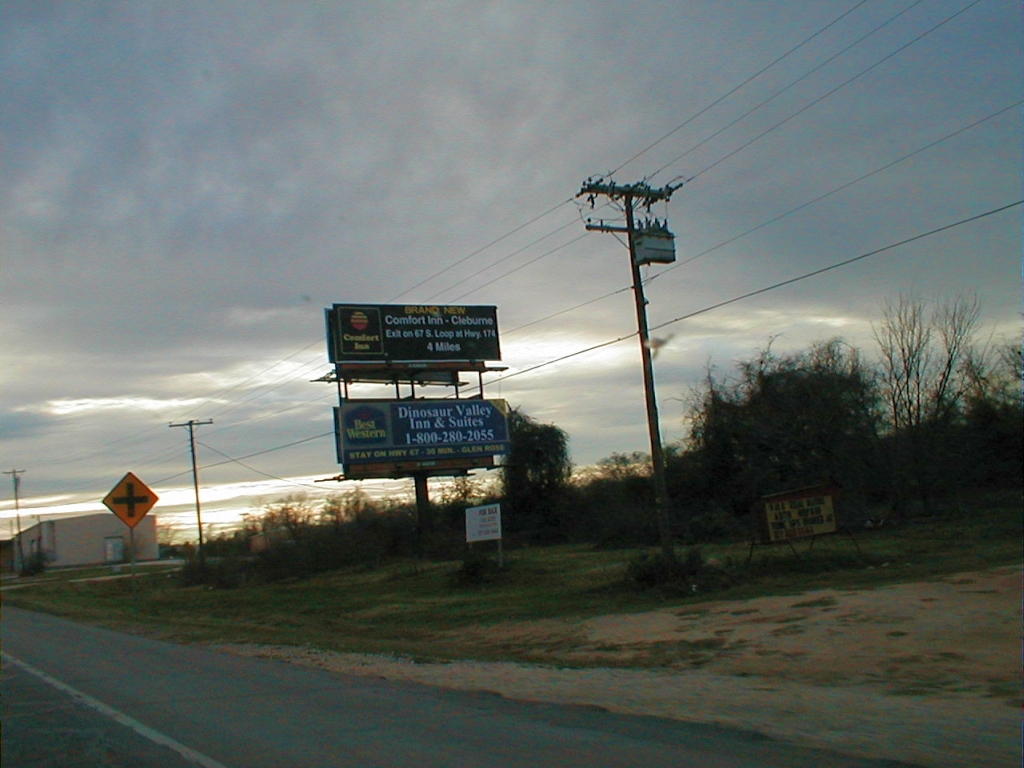In this photograph taken outdoors during sunset, a person travels along a light gray asphalt road with a faded white line in the bottom left corner. The sky is predominantly gray, featuring scattered white clouds with sunlight peeking through. The image is framed on the left by a road and a building, while power lines run across brown wooden poles lining this side. 

Prominently positioned in the middle of the image are two billboards. The top billboard advertises Comfort Inn, directing travelers to an exit, potentially Exit 67. Below this, the second billboard promotes Best Western and Dinosaur Valley Inn & Suites, including the contact number 1-800-280-2055. Adjacent to the billboards is a yellow intersection sign with a black arrow. 

On the right side of the image, a mixture of trees and a dirt area, possibly a dirt road or driveway, form the background. The scene captures a blend of natural and man-made elements, highlighting the journey amidst a serene yet transitioning sky.